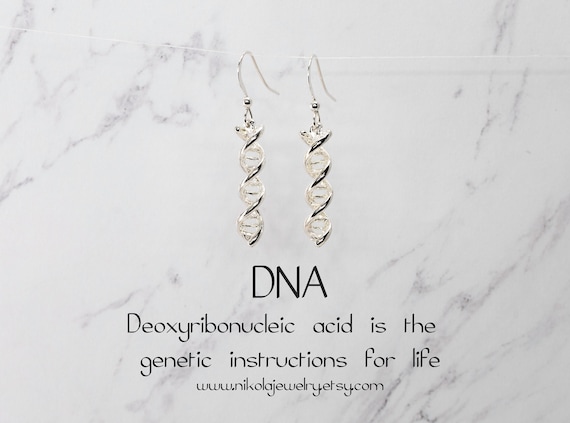This photograph showcases exquisite, silver DNA-shaped earrings that elegantly mimic the iconic double-helix structure. The earrings feature an S-like winding design, connecting two S-like shapes bridged by silver rods, creating an intricate and eye-catching pattern. At the top, each earring is secured by an eye hook adorned with smaller circular silver pieces, each set with a gem. The background resembles light gray marble with darker gray splotches, providing a sophisticated contrast to the earrings. Printed in bold black text beneath the earrings, the caption reads "DNA," followed by "deoxyribonucleic acid is the genetic instructions for life." The website www.nikolajewelrysetjewelryetsy.com is also included, guiding viewers to where they can purchase these unique pieces. Each earring, approximately two to two and a half inches long, is designed to be worn as a pair, making a beautiful addition to any jewelry collection.